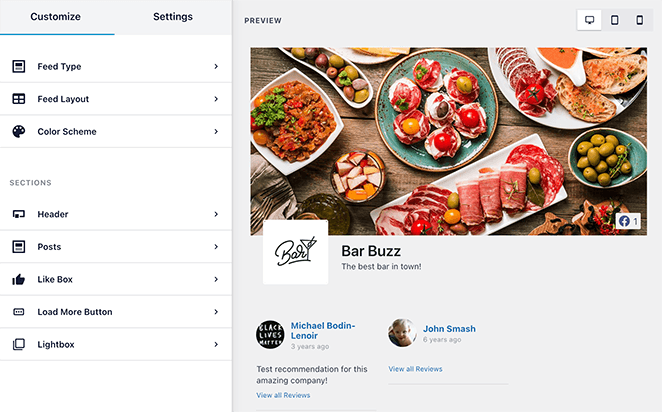The image depicts a webpage interface designed for customization settings. At the top left, the options "Customize" and "Settings" are displayed, with "Customize" underlined in blue, indicating it is the current selection. Below these options, the interface lists additional customization categories such as "Feed Type," "Feed Layout," and "Color Scheme," each accompanied by small illustrative icons.

Further down, a gray heading labeled "Sections" introduces a list of customizable sections, including "Header," "Posts," "Like Box," "Load More Button," and another "Like Box," each also marked with corresponding icons. All these items have right-pointing arrows, likely indicating that they are expandable or lead to further options.

On the right side of the interface, a larger section titled "Preview" occupies the top portion. At the top right of this section, different device format icons (desktop, mobile, tablet) are displayed, with the desktop icon highlighted. Below these icons, a preview image shows an inviting spread of various dishes, including olives, pink meat, a chili dish, and bread, all presented on white and blue plates against a wooden background. Beneath the image, the text "Barba is the best bar in town" is followed by names "Michael Bowden-Lenoir" and "John Smash," alongside their profile pictures.